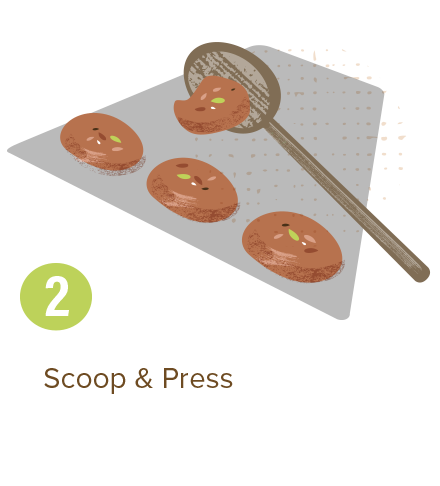The image depicts a cartoon-style, instructive clipart showing a grayish cookie sheet or parchment paper with four round, disc-like items that appear to be cookies, given the context and the accompanying text. Three of these cookies, which are brownish with yellow spots suggesting nuts or chips, are laid flat on the surface, while a spoon or spatula is shown placing a fourth cookie onto the sheet. Below the cookie sheet, the number "2" is displayed in white within a green circle, next to the instructive words "scoop and press" in brown text, emphasizing the action being performed in the image.